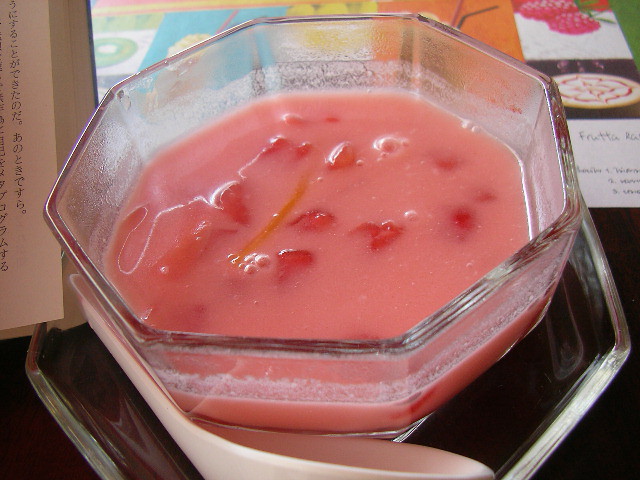The image features an octagon-shaped, clear glass container, resembling a blender jar, half-filled with a pink liquid, possibly a smoothie. Floating within the liquid are numerous red chunks, likely strawberries or cherries, along with a single yellow strip, potentially an orange rind. Adjacent to the container lies a small white scoop on a table. The tabletop showcases a colorful placemat adorned with various artworks and a table setting, including a glass. On the far left side of the table, there is a vertical strip of white paper with blue Asian writing on it.